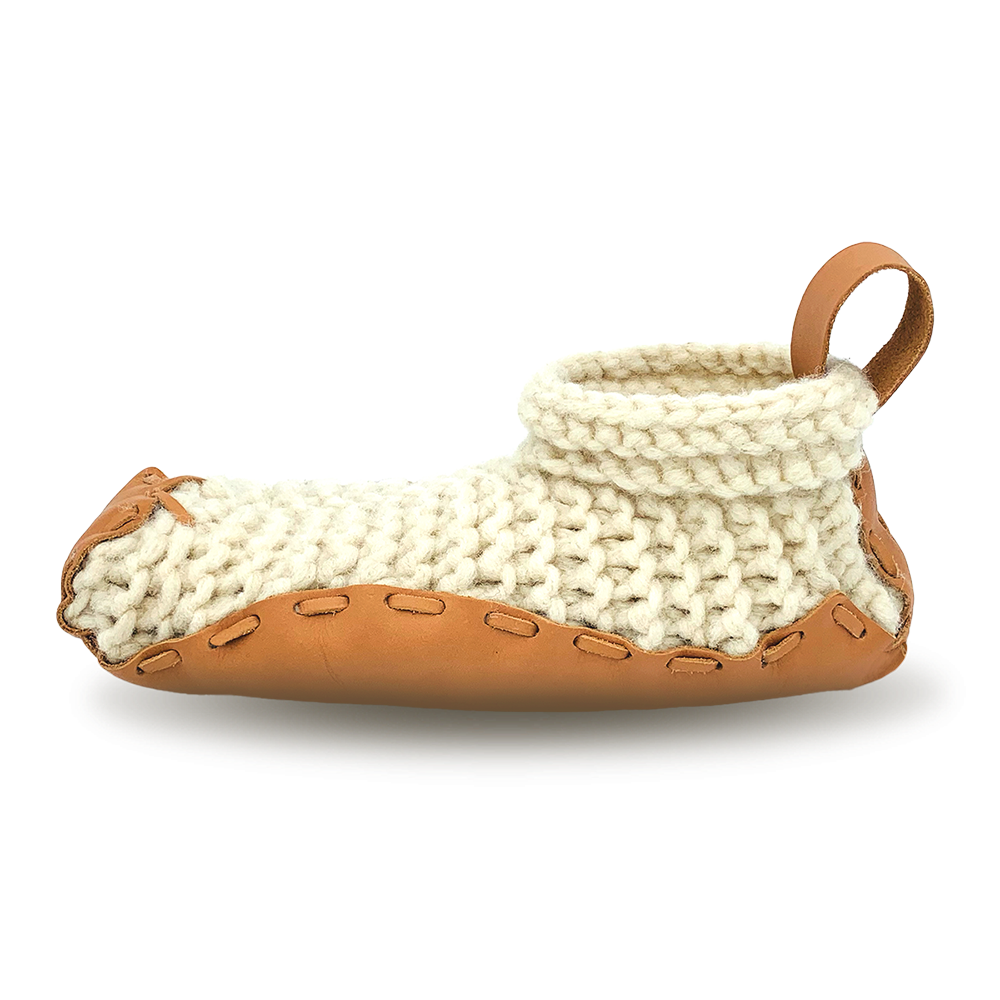In the white-background image, we see a beautiful handmade moccasin, oriented from left to right, showcasing its unique blend of materials and craftsmanship. The moccasin features a crocheted upper portion in a whitish-brown, cream color with intricate knotting. The base of the shoe, including the sole, toe, and heel, is crafted from light brown leather. This leather ascends the heel and wraps around the back, creating an extension that loops through a hole in the upper part of the shoe, forming a handhold. Additionally, the leather at the toe curves upward in a wave-like pattern. The leather sole is meticulously stitched to the crocheted upper through eyelets along the binding, employing ecru-colored, chunky, symmetrical stitching that highlights the detailed construction of this hybrid moccasin.